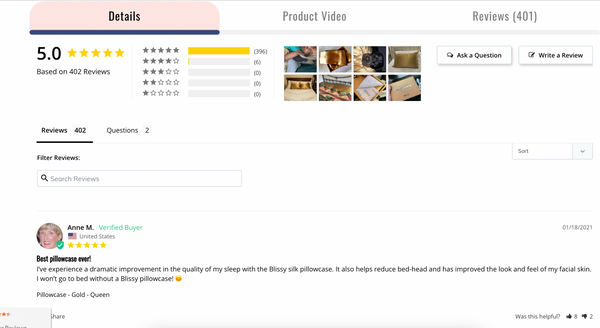This detailed caption describes an image showing a product review interface:

The screenshot captures a detailed view of a product review page. The product itself isn't clearly visible due to the small size of the accompanying images, which include four pictures across the top and four more below them. 

On the upper left-hand side, there is a section labeled "Details" in black text, set against a pink button background, with a dark blue line underneath. In the middle of the interface, gray text reads "product video." To the right of this, there's a "Reviews" section showing "401" written within parentheses.

Beneath the "Details" button, a 5.0-star rating is prominently displayed, with five yellow stars fully illuminated. Below this, the text states that the rating is "based on 402 reviews." To the right, there is a summary of all the reviews, indicating that a majority have four stars or more, as the lines for three, two, and one-star reviews are not filled.

To the right of the "Reviews (401)" section, there are buttons labeled "Ask a Question" and "Write a Review." On the left, under the "Reviews" heading, it notes "402 reviews" and "2 questions." A progress line is shown underneath the "402 reviews" section.

Below this, there is a "Filter reviews" label alongside a "Search reviews" search bar. To the far right of the search bar is a light gray "Sort" button with a downward-pointing arrow.

The first review is by Ann M., identified as a verified buyer with a turquoise icon. Her profile picture and a United States flag are displayed next to her name. She has given a five-star rating and titled her review, "Best pillowcase ever," in bold black text. Dated January 18, 2021, Ann's review praises the Blissy Silk pillowcase for dramatically improving her sleep quality, reducing bedhead, and enhancing her facial skin's appearance. She emphatically states she won't go to bed without a Blissy pillowcase, followed by a smiley icon. Beneath her review, it is mentioned that she reviewed a "Pillowcase Gold Queen."

In the lower left corner, a text snippet is unreadable. To the right is an engagement summary asking, "Was this helpful?" with thumbs-up and thumbs-down icons. The response indicates eight thumbs up and two thumbs down, though the text is quite small.